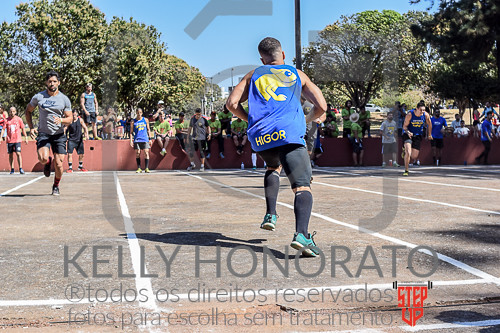This image captures a lively athletic contest featuring multiple contestants in action, running back and forth on a court divided by chalk lines. The participants, all dressed in athletic clothing, are focused on their respective lanes, which are separated by white markings on a brownish-gray surface. 

Dominating the scene is a male athlete in athletic shoes, long black socks, and a blue tank top emblazoned with a yellow chameleon and the name "HIGOR" in yellow text at the bottom. Adjacent to him, another contestant is seen wearing a similarly designed athletic shirt. The most clearly visible athlete, seen from the backside, is amidst a group of competitors in varied colored shirts, all engaged in the vigorous activity of the contest.

In the image's bottom right corner, the phrase "Step Up" in red text is prominent, accompanied by a barbell graphic above it. Additionally, the watermark "Kelly Honorato" appears in gray text, along with the words "are todos os derechos reservados fotos para escojas en tratamento" in the same style, suggesting attribution and rights information. In the background, several individuals can be seen either standing or sitting on a striking red wall, further emphasizing the dynamic and energetic atmosphere of the event.